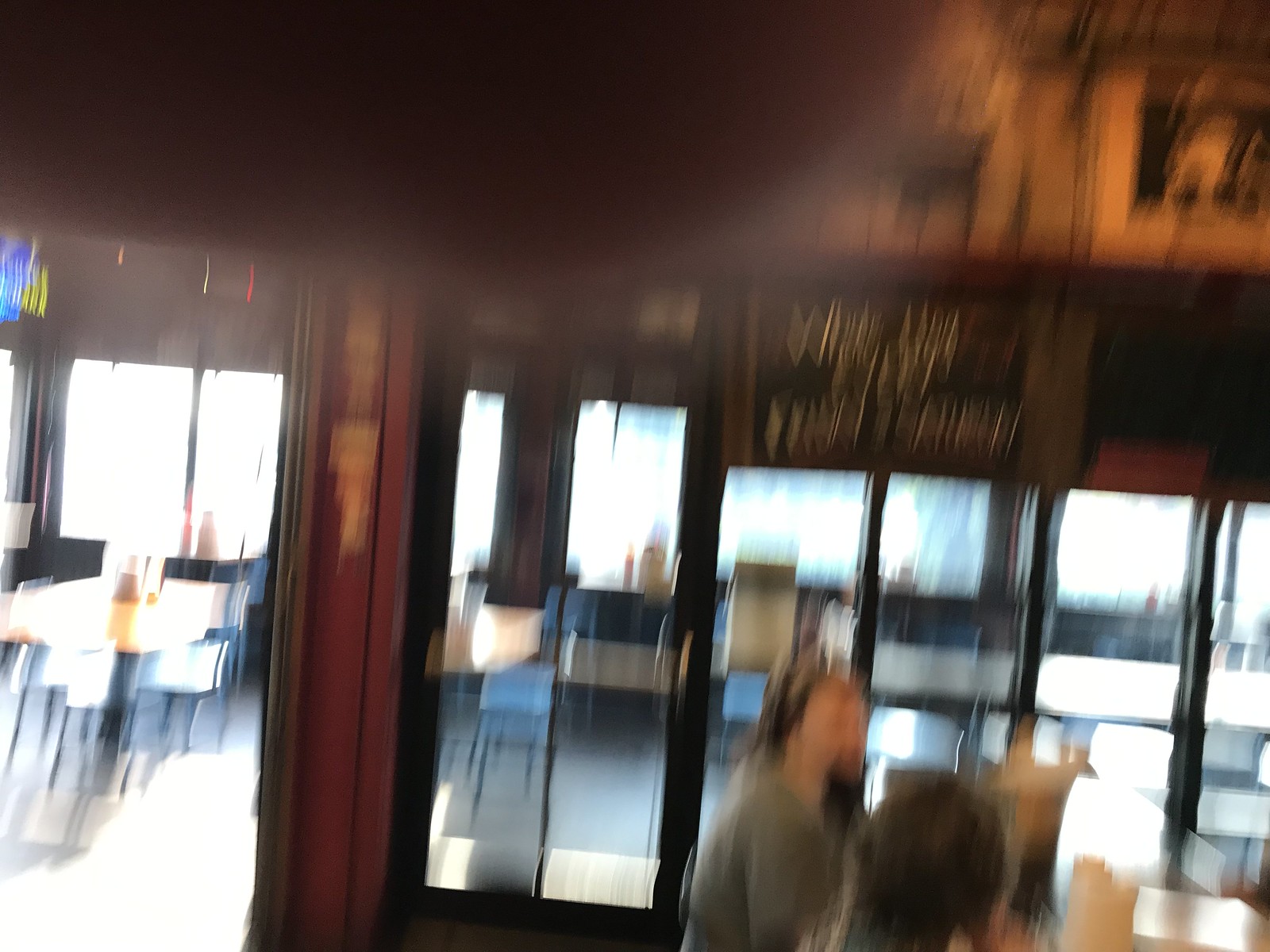This image captures a bustling restaurant scene, viewed from a higher vantage point that suggests the photo was either taken by a standing individual or a security camera. The perspective is elevated, providing an overview of the bar area. The photograph appears to be slightly out of focus and stretched, adding a sense of movement or distortion. 

In the left part of the image, there are two people seated at the bar. One person, positioned in the foreground, has their back to the camera, offering a clear view of the back of their head. The second person, further back, is facing the first individual, engaged in conversation or simply sharing their company. 

The background is lined with wood paneling and features glass elements, adding a touch of sophistication to the setting. Towards the right, two wooden doors can be seen, leading to what appears to be another part of the restaurant. There is also a doorway on the left. The background is populated with tables, both in the main room and a separate room beyond, which also has doors leading out. This adjacent room is similarly lined with glass windows, allowing natural light to permeate the space and contributing to an airy, open atmosphere.